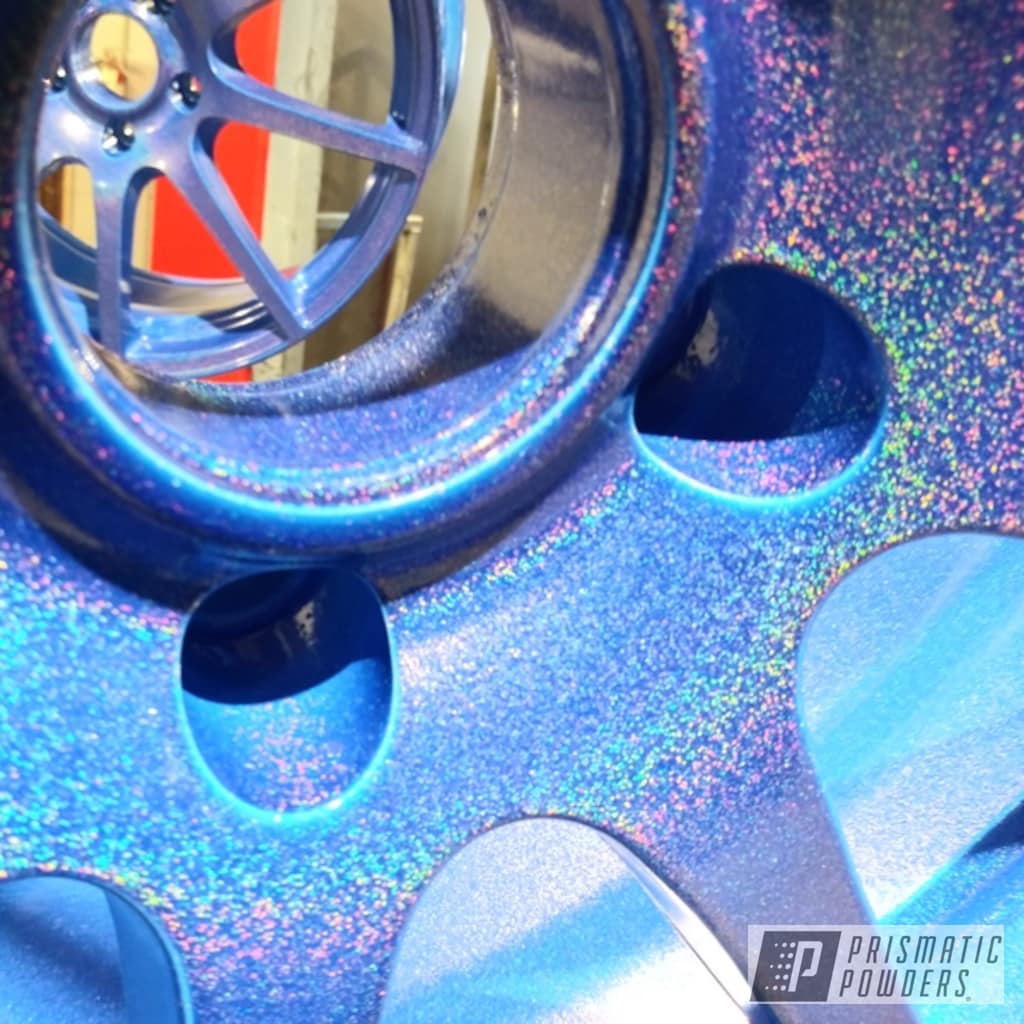The image features a close-up of a car wheel, prominently coated with prismatic powders, as indicated by the labeling in the lower right corner, which includes the prismatic powders logo, a "P" in a black box with dots. The wheel exhibits a main color of speckled, textured, light blue with iridescent qualities, displaying an array of lighter blue, pink, yellow, and teal flakes that shift in appearance depending on the lighting. This prismatic effect gives the wheel a grainy, multicolored look. The wheel's design includes a central hub and radiating spokes, and the background hints at another similarly painted wheel. The image seems to serve as an advertisement for prismatic powders, showcasing their vibrant, shifting paint effects on vehicle wheels.